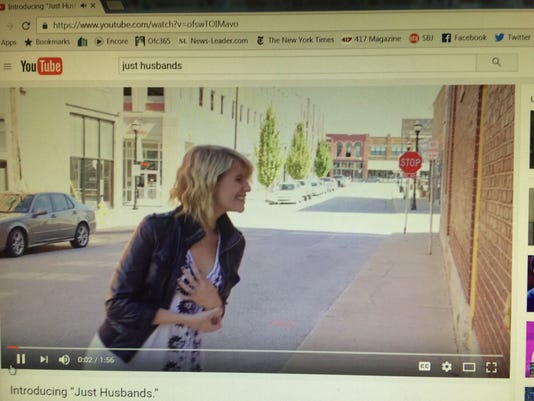This image is a detailed screenshot of a computer screen displaying a YouTube video. The browser's address bar shows the search term "Just Husbands," and the video is paused at the two-second mark of its total 1 minute and 56 seconds length. The freeze frame captures a young, smiling white woman with short, chin-length wavy blonde hair. She is dressed in a black leather bomber jacket over a white ornate blouse and stands on an urban sidewalk adjacent to small brick buildings that resemble restaurants with canopies. The street scene features a silver car approaching from the left, a visible stop sign, and another parked vehicle. Additionally, the video description under the image reads "Introducing Just Husbands" in black text. The overall scene suggests a cheerful moment captured in an urban downtown setting. All visual elements in the screenshot, such as the browser's bookmarks and the video frame, are upright and properly oriented.